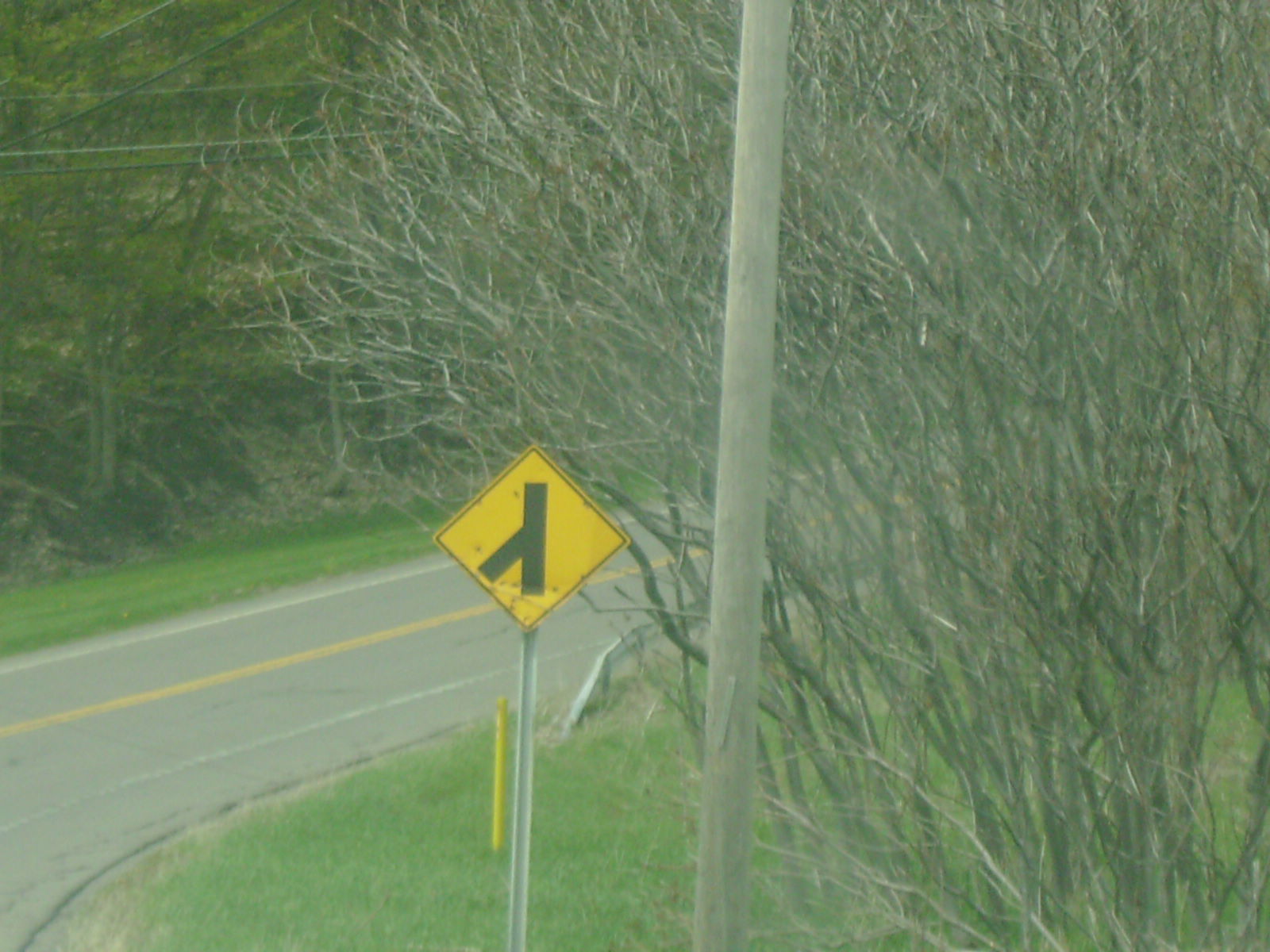This image captures a gloomy, overcast day, featuring a winding road cutting through a grassy field. On the right side of the image, leafless trees with thick, barren branches stretch toward the sky. The center of the image is dominated by a tall utility pole or light pole, its top extending beyond view. Near the center-left edge of the image, a prominent, square-shaped (diamond-positioned) yellow traffic sign on a metallic pole with a black "Y" or "V" pattern indicates an upcoming merge. Adjacent to this sign, a shorter yellow pole is anchored in the ground beside a metal guardrail. The asphalt road curves from the bottom left to the middle right, marked by a central yellow line and flanked by white side lines. Surrounding the road is lush green grass, interspersed with bushes, some bearing leaves and others not, emphasizing the somber and transitional nature of the scenery.